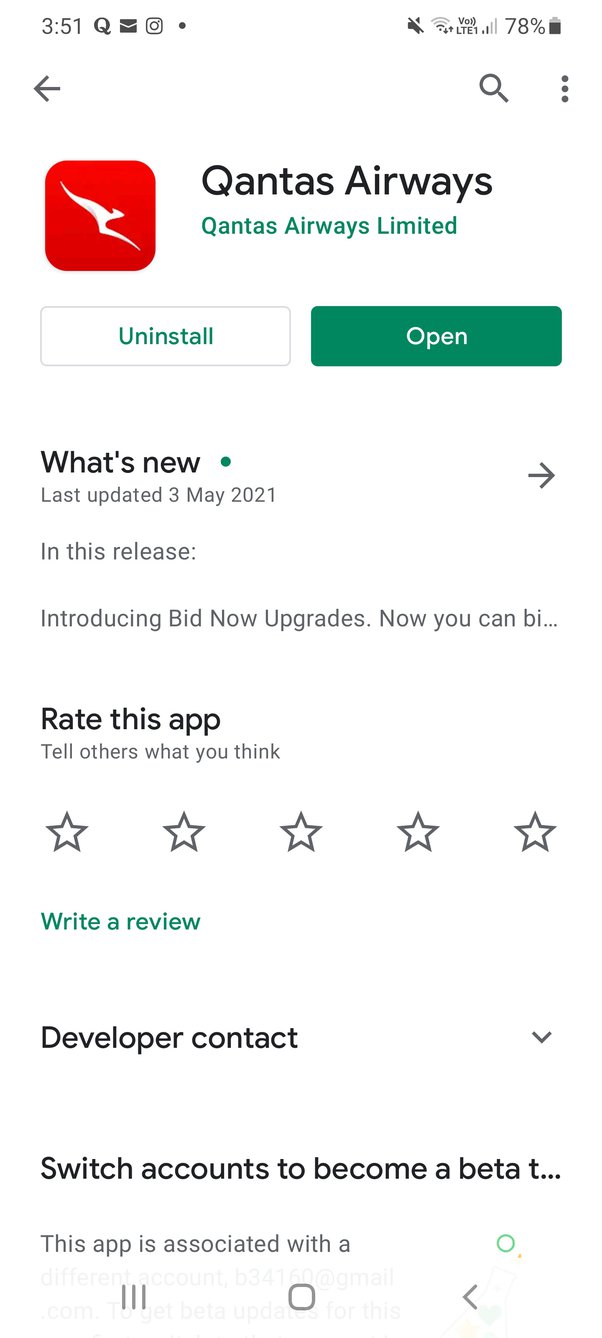This is a detailed screenshot showing the Qantas Airways Limited app as viewed in an app marketplace. The top section of the screen displays the system status icons including the time (3:51), a queue for notifications (likely from Quora), an envelope for email, the Instagram icon, a muted alert sound, one bar of Wi-Fi indicating LTE connectivity, two bars for cellular signal strength, and a battery percentage at 78%. The navigation elements on top include a back arrow, a search magnifying glass, and a three vertical dot menu on the right.

Prominently, the icon for the Qantas Airways app is a red square with rounded corners featuring a sleek, white kangaroo. Underneath the logo, in large black text, it reads "Qantas Airways," and in smaller green text, "Qantas Airways Limited." Below these, there are two interactive buttons: a white 'uninstall' button with green text and a gray border on the left, and a green 'open' button with white text on the right.

The 'What's New' section follows, marked with a green dot and the last update date, "May 3rd, 2021." It includes a brief message about new features: "Introducing bid now upgrades. Now you can bi..." though it gets cut off. Below this, bold text invites users to "Rate this app, tell us what you think," followed by five empty stars and a 'write a report' option in green text.

Further down, there's an expandable 'developer contact' section with a drop-down arrow. Beneath that, another bold text section reads, "Switch accounts to become a beta..." but the text is truncated.

Finally, at the very bottom, there's a note indicating this app is associated with something unspecified, alongside a simple navigation menu.